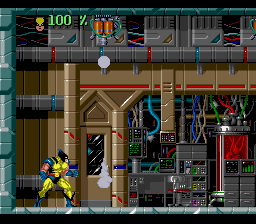This is a detailed screenshot from the video game "Wolverine: Adamantium Rage" on the Super Nintendo. The image depicts Wolverine in a setting that resembles a scientific laboratory. The top left corner displays his health, which is at 100%, indicated by a green bar beside a small icon of Wolverine's face. The laboratory background features a mix of goldish-brown hues and elaborate details, such as computer dials, green and red lights, and various cords, suggesting an advanced technological environment. Wolverine, the central character, is positioned to the left of the frame. He is depicted as a muscular figure wearing a light green outfit with blue gloves, blue boots, and a black helmet. Highlights of yellow accentuate his pants and shirt, with a red stripe on his arms. The composition suggests it is the start of a level within the game. The left vertical section and top horizontal section of the image are framed by a green border. Wolverine is seen moving towards the machinery-filled area on the right, enhancing the impression of an immersive computer or scientific room setting.